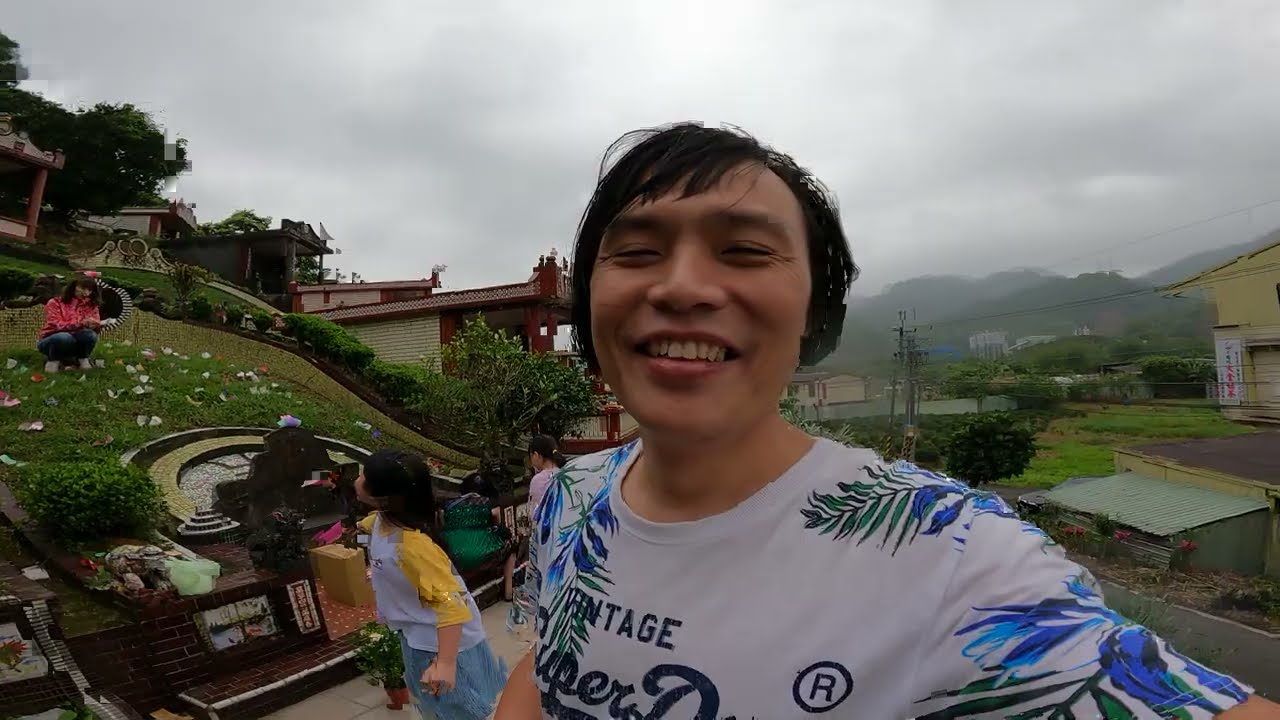The photograph is an outdoor selfie featuring a young Asian man, a woman, and a child, all smiling and appearing to enjoy their time together. The man, centrally positioned, has short black hair and wears a distinctive white shirt adorned with blue and green floral designs and text. To his left, a woman with long black hair crouches on a grassy knoll near a steep hill decorated with numerous flowers. The child, dressed in a yellow and blue top and blue bottoms, stands to his left. In the background, an overcast sky looms over a mist-covered landscape featuring greenery, hills, and distant mountains. A yellow building with a large green dumpster is visible to the right of the man, while a shrine, with a turtle statue next to it, sits atop the flower-covered hill. The image captures a moment of joy and togetherness amidst a scenic and somewhat mysterious setting.